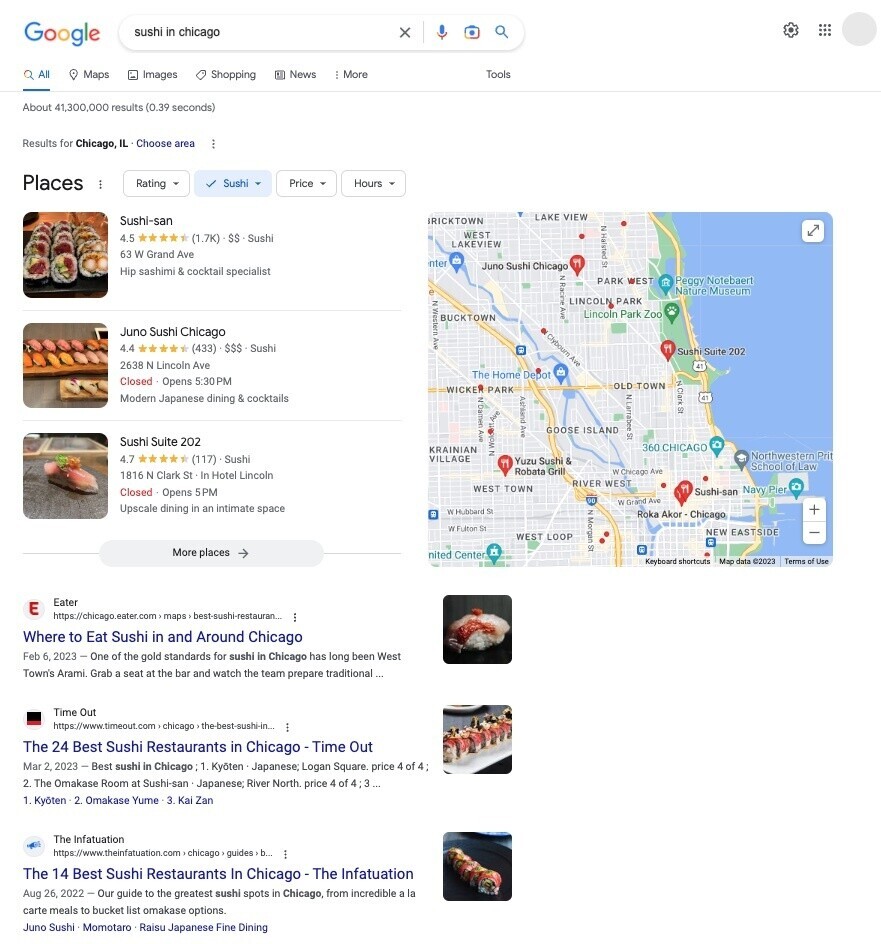The image features a Google search results page on a pristine white background. In the top left corner, the distinct Google logo is present with a search box next to it containing the query "sushi in Chicago." On the left side, a bold black font section titled "Places" lists three entries. 

The first entry includes a vertical rectangular image of sushi rolls. To the right of this image, the place is named "Sushi-san," followed by a rating of 4.5 with four out of five stars highlighted in yellow. It is noted that there are 1.7K reviews. The restaurant is marked with two dollar signs, indicating moderate pricing, and it is categorized under sushi. Beneath the name, the address is provided as 63 West Grand Avenue with a brief description: "Hip sashimi and cocktail specialist."

The second entry is for "Juno Sushi Chicago," and the third lists "Sushi Suite 202," both following the same format with accompanying vertical rectangular images and detailed information.

On the right side, there is a map pinpointed with red teardrop markers symbolizing dining locations, each marked with a fork and knife icon. 

Further down in the center of the screen, a horizontal rectangular button labeled "More places" in black font directs to additional entries. Below this, additional search results are displayed. The first result is from Eater, with an “E” logo on the left and text in blue font reading "Where to eat sushi in and around Chicago." A vertical image accompanies this entry, alongside the date February 6, 2023, and a brief description highlighting West Town's Armani as a gold standard for sushi in Chicago with a recommendation to watch the team prepare traditional dishes.

The second result is from TimeOut, titled "The 24 best sushi restaurants in Chicago - TimeOut," and the third is from Infatuation, titled "The 14 best sushi restaurants in Chicago - Infatuation," each with similar formatting featuring vertical images and headlines.